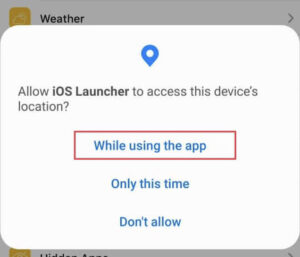The image showcases a pop-up window overlaying a grayed-out background, with the top part of the original screen faintly visible. The visible part at the top displays the text "Weather" in black font, alongside a yellow square with an indistinct white logo. A gray arrow pointing to the right appears in the upper right-hand section.

The pop-up window has softly rounded edges and stands out against the background with its white color. At the top center of this pop-up box is a blue "ping" icon. Below this icon, the text reads: "Allow iOS Launcher to access this device's location." Beneath this prompt, three options are listed for the user to choose from: "While Using the App" at the top, followed by "Only This Time," and finally, "Don't Allow" at the bottom. The overall design is clean and focused, guiding the user’s attention towards making a selection.